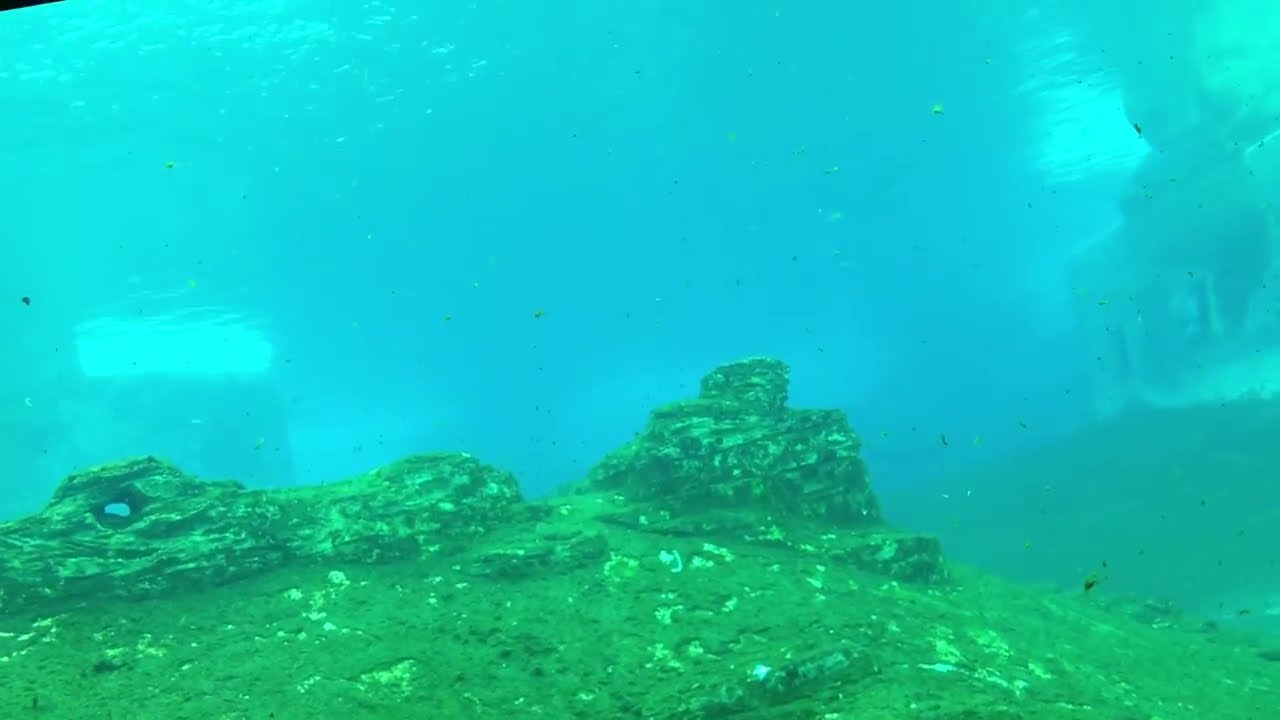This is a horizontally aligned, rectangular underwater photograph capturing a vibrant marine scene. The upper half of the image showcases a beautiful gradient of blue hues with patches of light green, indicative of sunlight filtering through the water. Bubbles can be seen at the top, hinting at the water's surface above. The lower half features a textured ocean floor, predominantly brown and green with some white elements. The seafloor rises into a hill adorned with various rock formations. On the left side, one rock structure has a small hole in it, creating an interesting feature. Dominating the right side of the image, near the top, an indistinct white structure—possibly part of a boat—adds a touch of mystery. The entire scene is accented by the play of light and shadows dancing through the water, creating a serene and captivating underwater tableau.